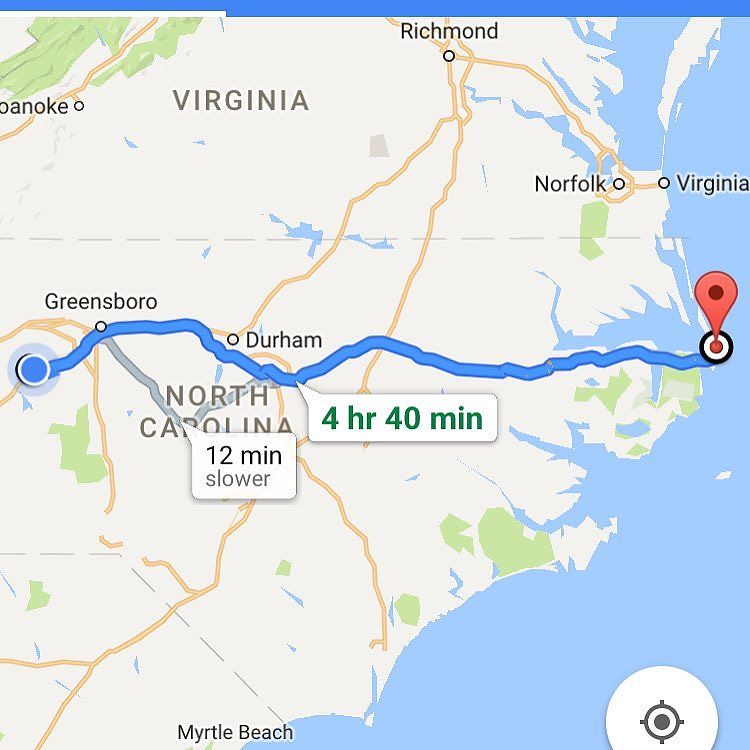This screenshot from Google Maps displays a detailed aerial view of a route starting from the coast of Virginia, near Norfolk, and traversing through the states of Virginia and North Carolina. The satellite imagery highlights the landscape from above, showcasing state borders and major highways. The designated route is marked in blue, beginning at a red "You are here" indicator on the coast of Virginia. It progresses southwest, passing through cities like Richmond, Virginia, and Durham, North Carolina, before reaching its terminus just past Greensboro, North Carolina. According to the map, the total travel time is approximately four hours and forty minutes. An alternate route option is noted to be 12 minutes slower. The map also displays various other geographical markers and city names, including the area of Onancock in Virginia.